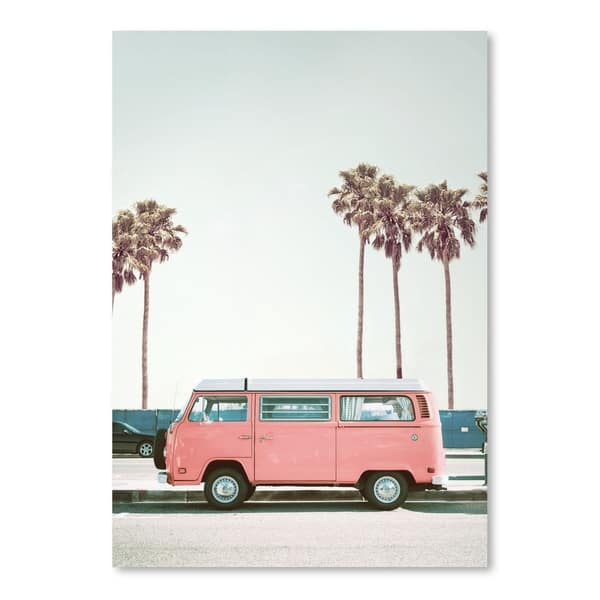This photograph showcases a retro 1960s-style van parked on the left side of a light gray road. The van, a striking pink with a white roof, is prominently positioned in the image. We see its side profile, revealing three windows: the rear window adorned with white curtains, the middle window with silver stripes, and the front window which appears ordinary. The black tires with aluminum rims add to its vintage charm. In the background, a blue-green wall stands alongside a compound wall, complemented by the serene presence of tall palm trees with lush green fronds against a transitioning pale blue to gray sky. The scene evokes a nostalgic atmosphere reminiscent of a bygone era.